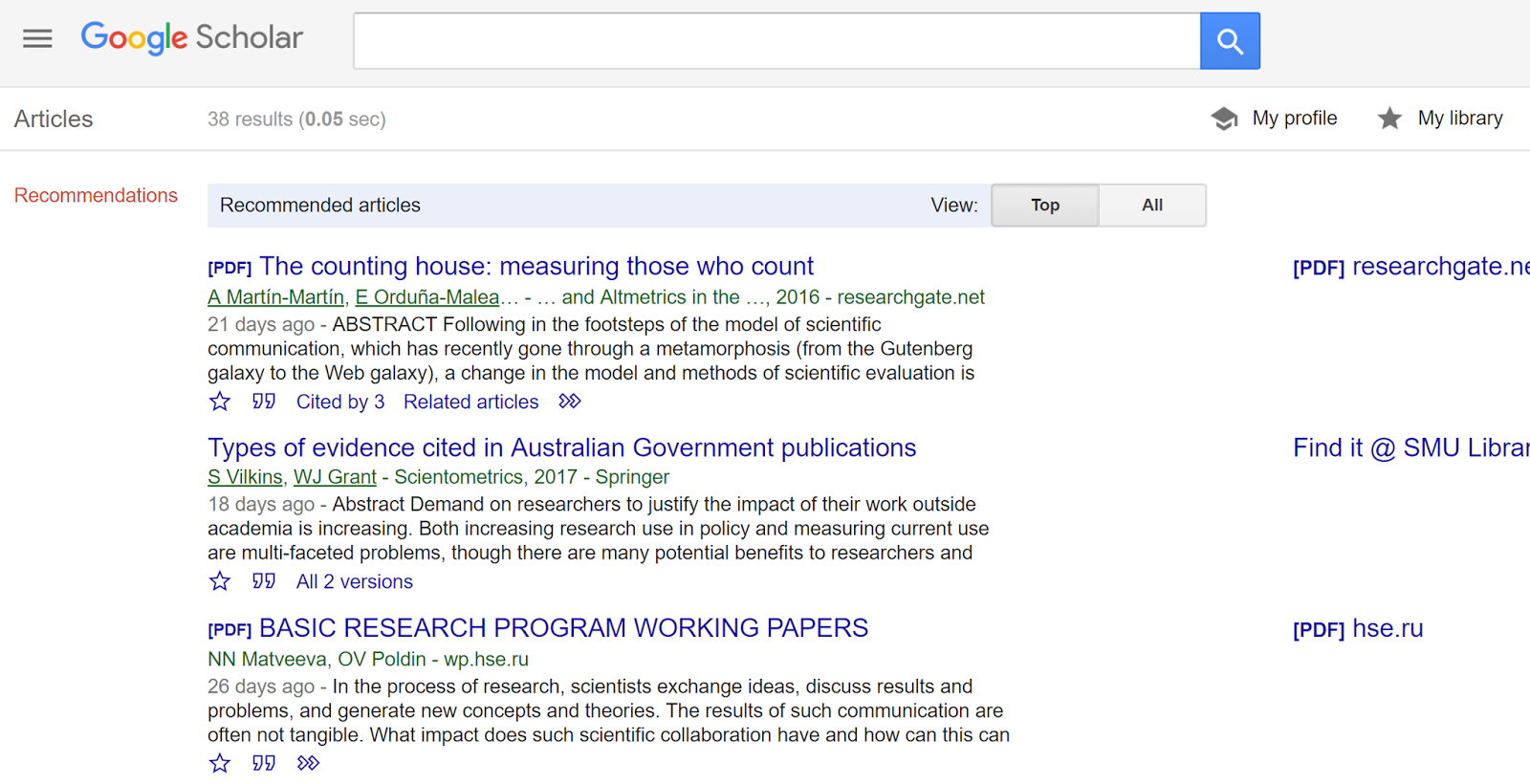This detailed screenshot from a Google Web Search interface illustrates several elements of a search results page. At the top, there is a blank URL field enclosed in a blue square, which features a white magnifying glass icon on its right side, signifying the search function. Underneath, there is a large white rectangle, representative of the main search area.

On the left-hand side of this area, the word "Articles" is displayed in black text, followed by a gray text indicating "38 results (0.05 seconds)." On the right-hand side, there is a black graduation cap icon next to "My Profile," both displayed in black text. Adjacent to that is a black star icon next to "My Library," also in black text.

Within the main white rectangle, there is another section labeled "Recommendations," written in red text on the left-hand side. Next to this label, a light blue rectangle can be seen, which features the text "Recommended Articles" in black on the left and "View..." on the right. This section contains two clickable buttons: the first button, shown in dark gray because it is selected, displays the word "Top" in blue at its center. The second button, in a lighter gray, also has blue text in the center, though the specific text is obscured.

On the far right, there is text enclosed in brackets reading "PDF," followed by the truncated text "ResearchGate...". Another entry reads "Find it at SMU Library," but this too is cut off. Similarly formatted entries follow, including one marked "PDF," reading "TheCountingHouse... Measuring Those Who Count." Subsequent entries are titled "Types of Evidence Cited in Australian Government Publications" and "PDF BASIC RESEARCH PROGRAM WORKING PAPERS," all written in hyperlinked blue text. 

The detailed visual elements and truncated excerpts suggest a rich array of search results primarily linked to scholarly articles and PDFs, providing a comprehensive overview of the search engine's academic resource offerings.